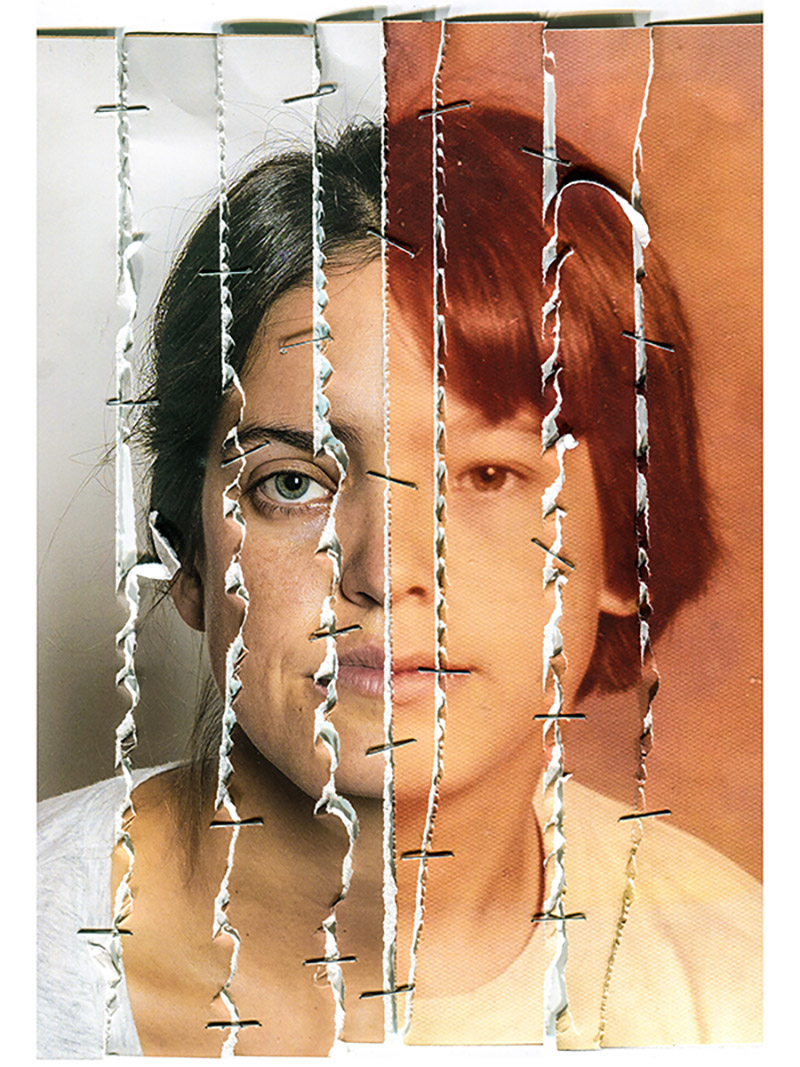The photograph depicts a composite image of a woman created from eight vertically torn strips. The left side of the image features four strips that are bright and possibly true to color, showing a woman with dark hair and greenish eyes wearing a white blouse. In contrast, the right side consists of four darker strips roughly stapled together, depicting a little girl with brown eyes. The central strips align the two faces well, merging them seamlessly. The overall composition suggests a haunting narrative, possibly indicating the passage of time, with the modern woman on the left transitioning to a younger version or an entirely different child on the right. This unsettling, artful presentation invites interpretations of loss, growth, and connection, as if reflecting on how two different moments in life or two related individuals are intertwined.